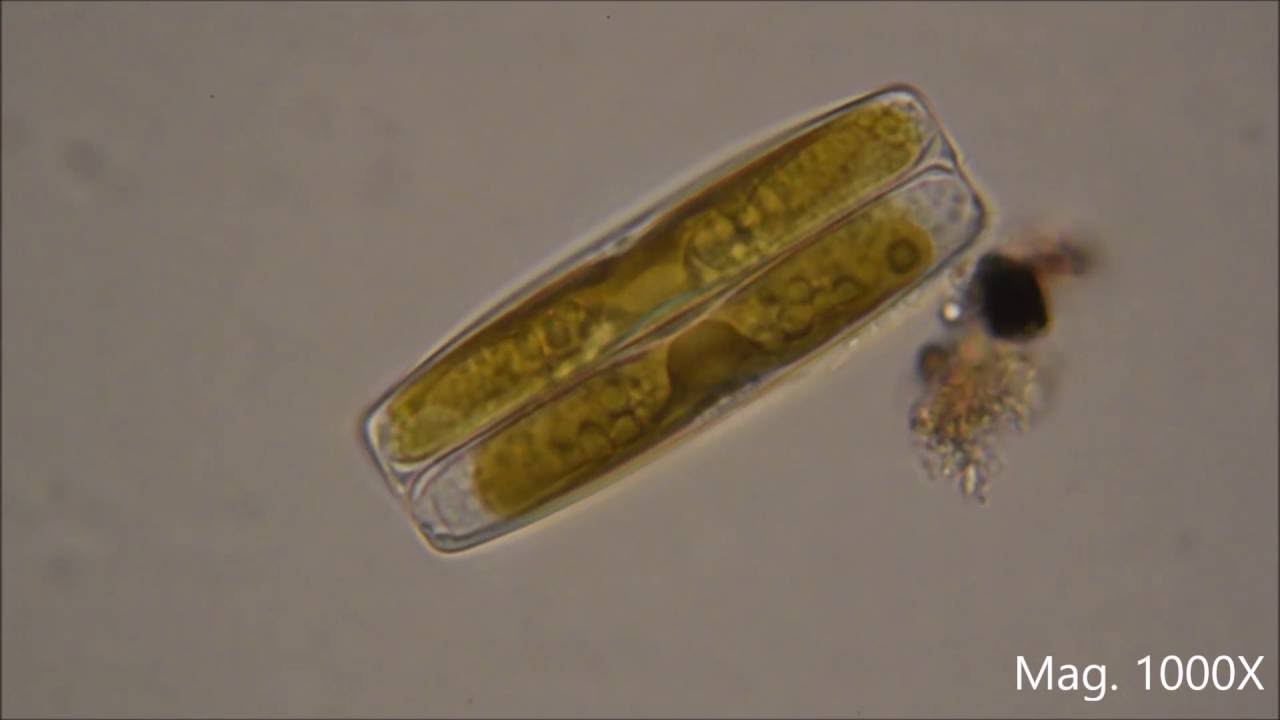The image is a micrograph, depicting a highly magnified object at 1,000 times magnification, as indicated by "MAG 1000X" at the bottom right corner. The main subject, centrally located, consists of two adjacent, semi-transparent, rectangular segments with varying shades of green and olive green liquid inside. These segments appear textured and contain multiple small, bubble-like circles. The background is a dark, splodged gray, contributing to the image's unprofessional feel. To the right of the main segments, there is a dark green, spindly structure with a small black dot beside it, adding to the detail and complexity of the micrograph.